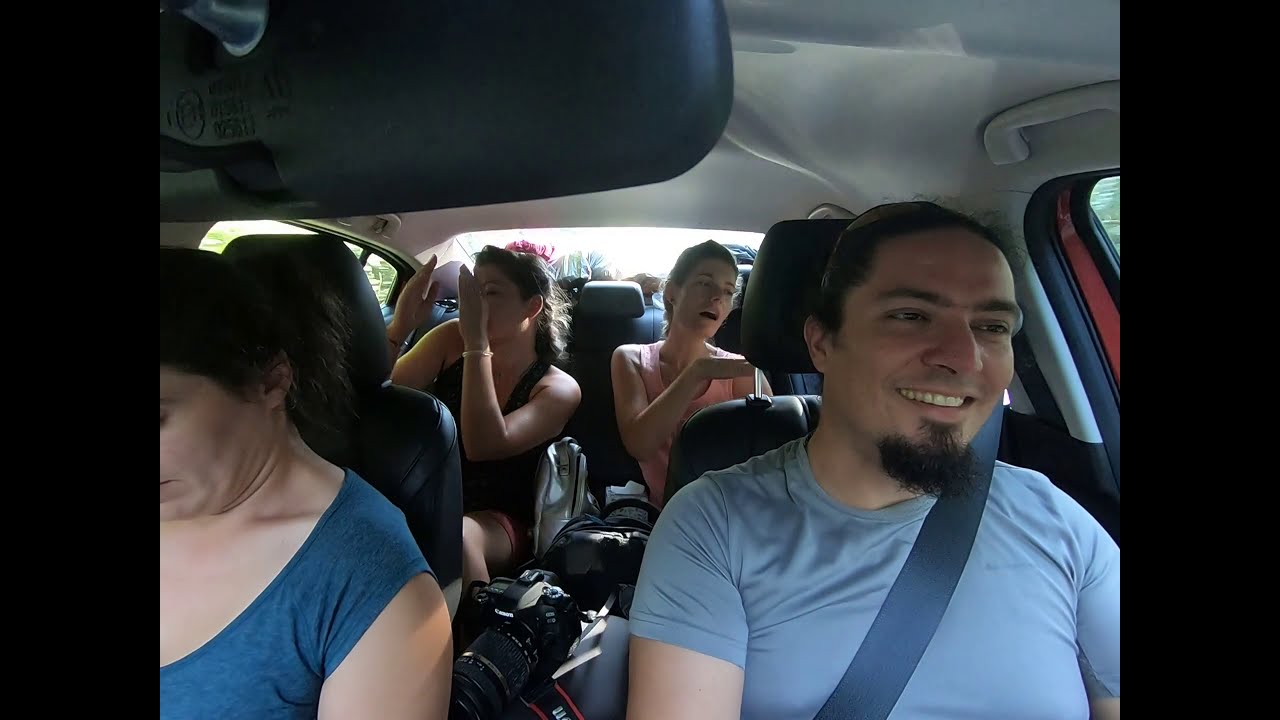The image depicts an interior view of a car from the windshield's perspective, revealing its diverse occupants and lively atmosphere. In the foreground, a man with dark hair and a black goatee is in the driver’s seat, clearly visible from his light blue, short-sleeved shirt and seatbelt crossing from his left shoulder. Beside him, a woman is wearing a blue v-neck top; her dark hair is partially visible as she glances downwards, and a black camera lies between them. The car's interior features dark seats with light gray upholstery on top, including a rearview mirror in the upper left-hand corner. Behind the front passengers, two young women occupy the back seats, both with dark hair. The woman on the left, dressed in a dark tank top with a hint of pink in her hair, appears to be clapping her hands. The woman on the right, wearing a pink tank top, is engaged in an enthusiastic gesture, possibly singing or talking, as suggested by her open mouth and dynamic arm movements. The exterior of the car is tinted a dark orange and the scene is framed by black bars on each side of the image.